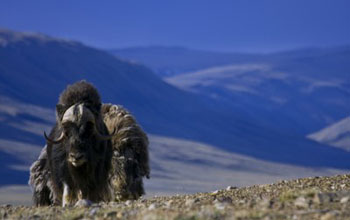In this rectangular outdoor photograph, two majestic buffalo (or bison) are captured standing side by side, with one noticeably in front of the other. The buffalo in the foreground is dark brown, facing forward, and features prominently curled horns or antlers emerging from the lower sides of its head. Its impressive frame includes a large hump covered in thick brown fur. Notably, the front legs or hooves of this buffalo display white markings. Behind this buffalo, another animal is visible, but from a rear view, appearing lighter in color. The scene extends to a distant landscape where rolling mountains shift in muted shades from darker gray to lighter white and blue hues. The upper fifth of the image showcases a clear blue sky, unmarred by clouds. The ground beneath the animals is a rough blend of rocks and dried grass, grounding the wild, natural setting of this photograph.